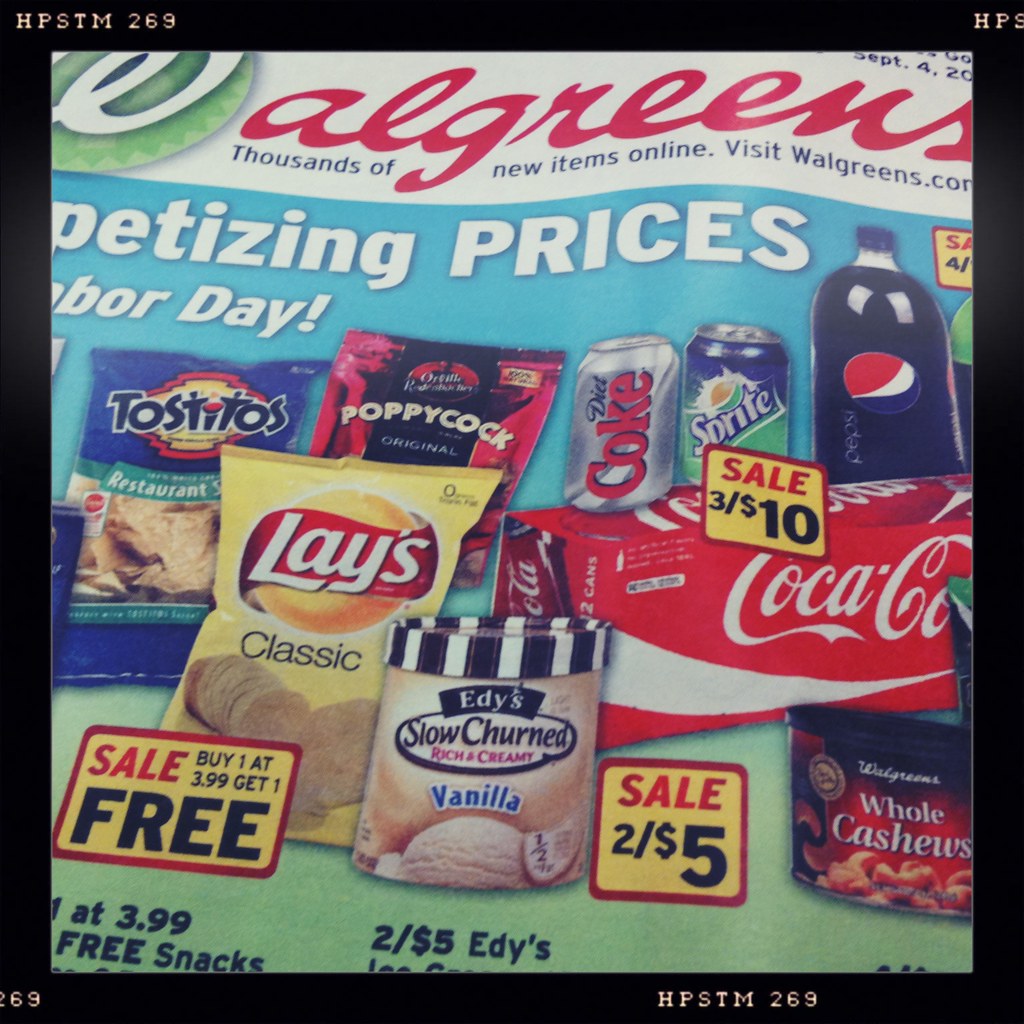The image features a Walgreens shopping insert prominently framed by a solid black border. The Walgreens logo, with its signature green circle and white "W," is highlighted against a red font. The insert, possibly part of a weekly circular for the US-based chain, showcases a variety of products on a blue background, indicating game day or holiday sales. Visible items include Tostitos chips, Poppycock snacks, Lay's Classic Potato Chips, Edy's Slow Churned Vanilla Ice Cream, Coca-Cola, Diet Coke, Pepsi, Sprite, and whole cashews. Yellow sale signs accentuate the discounts, suggesting these items are ideal for satisfying munchies. The colors in the advertisement range from black, white, yellow, red, blue, to various shades of brown and green. Additionally, a code noted as "HP STM 269" appears in the upper left and lower right corners of the insert.